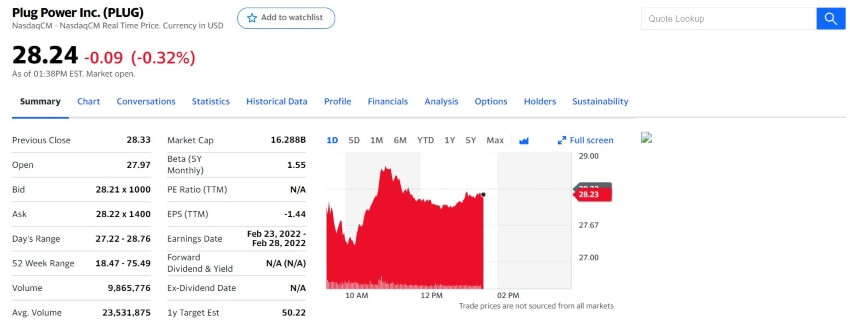The image displays a detailed financial overview of Plug Power Inc. in the upper left corner, with "Plug Power Inc (PLUG)" in black text followed by an option to click and add it to a watchlist. The current stock price is prominently shown as "28.24" in bold black text, indicating a slight decrease of "0.09" in red text (down 0.32%). The data is noted as being accurate as of 1:38 p.m. Eastern Time, with the market still open.

Below the main header, the interface features several subcategories, with "Summary" underlined and adjacent options including Chart, Conversations, Statistics, Historical Data, Profile, Financials, Analysis, Options, Holders, and Sustainability.

The red graph area beneath this summary plots the stock's performance over the day, marked with times from 10 a.m. to 2 p.m. The stock's price at 2 p.m. is highlighted in a red rectangle as "28.23." Along the top of the graph, multiple timeframe options are available (1M, 6M, YTD, 1Y, 5Y, Max), alongside navigational arrows and a "Full Screen" option in blue. To the left of the graph, additional information such as average volume, current volume, and the upcoming earnings dates (February 23, 2022 - February 28, 2022) is noted.